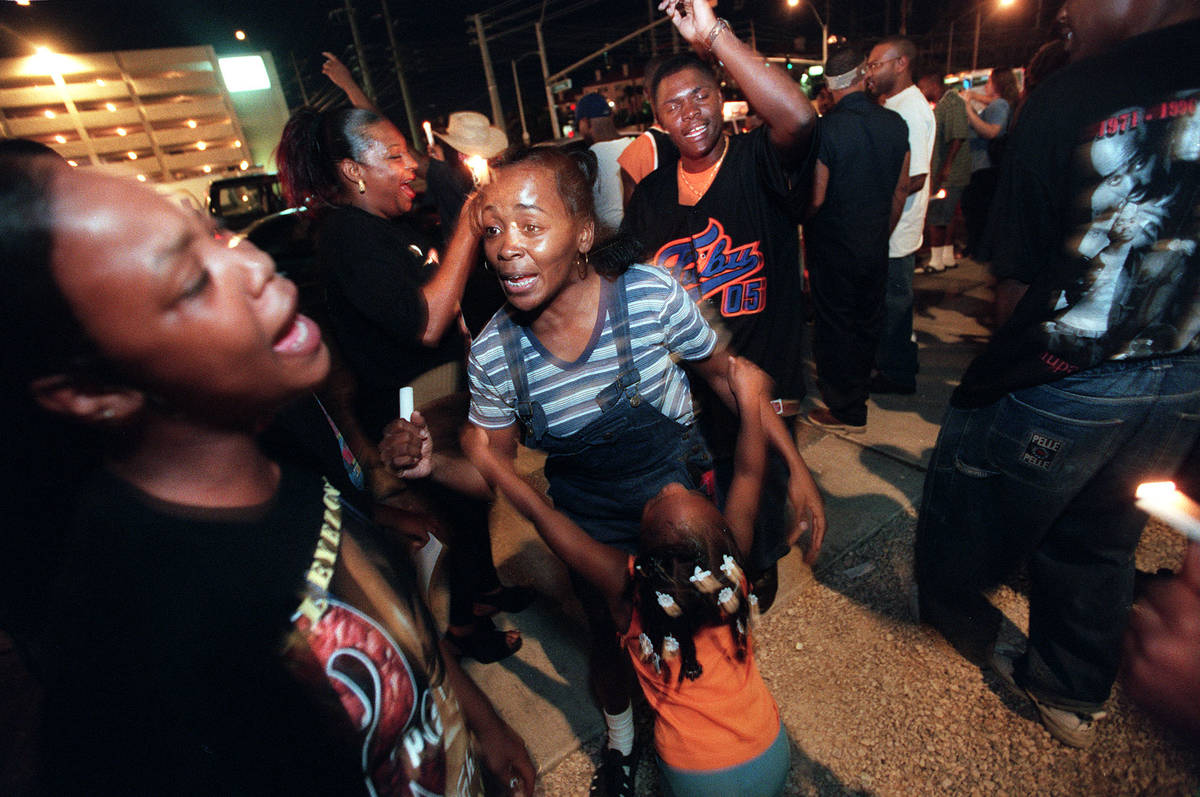In this nighttime image, a group of African-American individuals, including men, women, and children, are gathered on a gravel and concrete area in front of a five or six-story parking garage. The scene suggests a lively or possibly tense outdoor event, with people appearing agitated or excited. The central figure is a middle-aged woman wearing short overalls and a blue striped short-sleeved shirt. She holds a short white stick in her right hand and is engaged with a young girl, approximately 4 or 5 years old, wearing an orange top and gray bottoms. The girl, with braided hair adorned with trinkets, has her hands on the woman's arms and looks up at her. 

To the left, another woman with an open mouth and a black t-shirt with yellow lettering can be seen, her expression directed to the right. Just behind her is a young African-American man wearing a sports jersey, seemingly yelling. On the right side of the image, partially captured, is another man in a black shirt with an image and red numbers reading "1971 to 1996." He is walking towards an additional group of people, including a white woman and more African-American men, some of whom are holding candles. In the background, there are streetlights, poles, and a slatted wood wall, hinting at an urban setting. The lighting is coming from the far left and above overhead, adding to the dramatic ambiance of this potentially historical or protest scene.